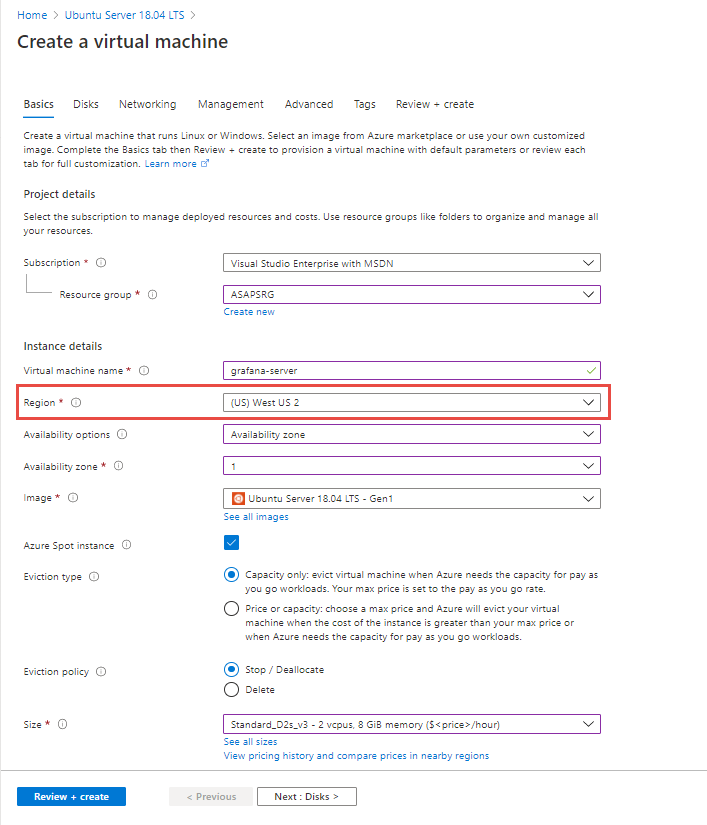Here is the cleaned-up and detailed caption for the image:

"The image displays a page from the Azure portal interface focused on creating a virtual machine. Several tabs are visible at the top, including Disks, Networking, Management, Advanced, Tags, and Windows. The instructions advise users to either select an image from the Azure Marketplace or upload their customized image. After completing the Basics tab, users can either proceed directly to 'Review + Create' to provision a virtual machine with default parameters or review each tab to fully customize the virtual machine settings."